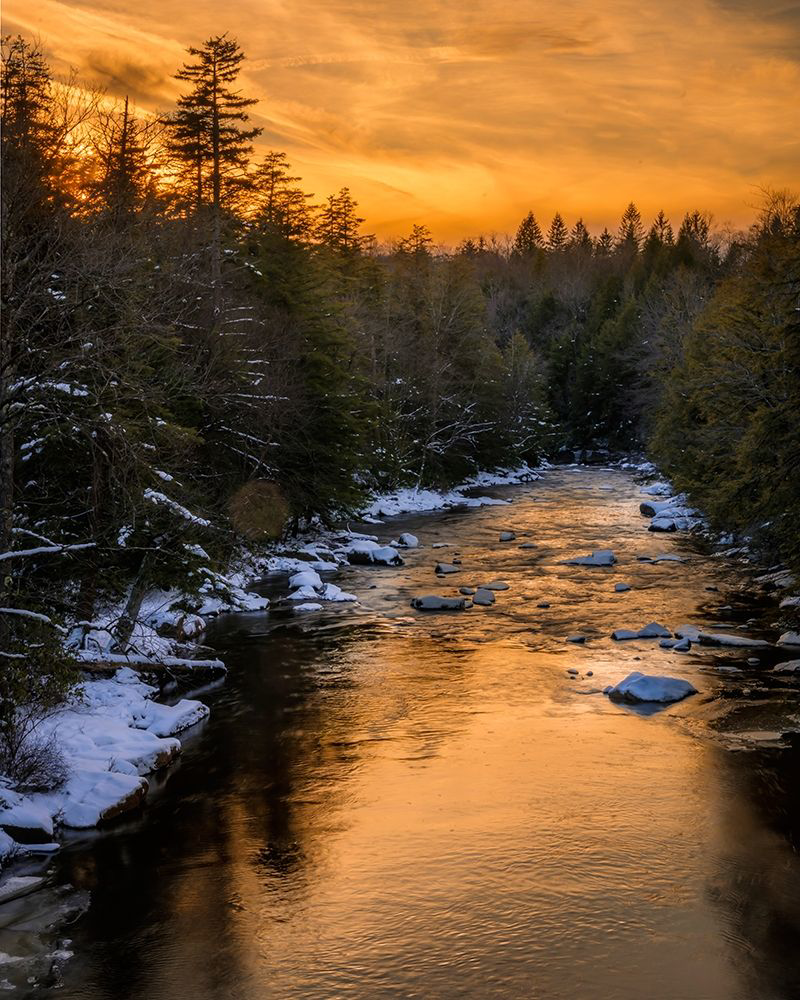This is a detailed outdoor photograph taken during the daytime, capturing a serene, narrow river flowing through a picturesque winter landscape. The river, shallow with visible rocks, reflects the vibrant orange hues of an evening sky interspersed with wisps of gray clouds. Along the banks, snow-covered rocks and land frame the water, which flows gently towards a distant expanse of tall, dense evergreen trees. Among the trees, a mix of snow-clad firs and bare deciduous trees can be seen, their green and white contrast beautifully with the wintry setting. The scene is serene and tranquil, enhanced by the reflective orange and gray tones in the river, echoing the sky's brilliant colors.